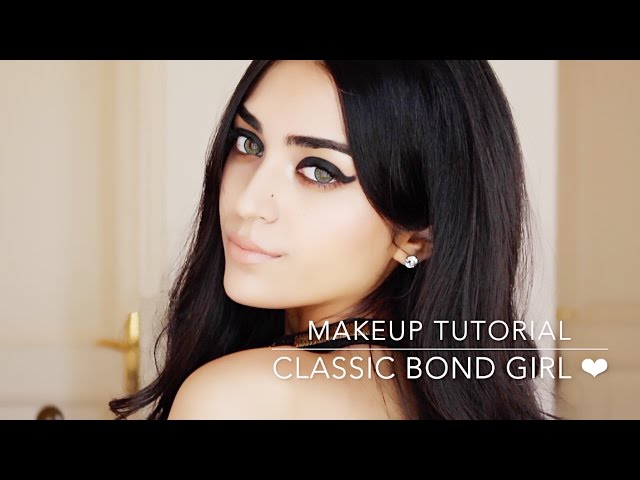This image, suitable for a magazine or social media tutorial, captures an elegantly styled woman epitomizing a "Classic Bond Girl." She poses with her face turned towards the camera, showcasing her intricate makeup. She has striking deep green eyes, accentuated with thick black eyeliner in a cat-eye design that wings out at the edges. Her eyebrows are perfectly shaped and darkly lined. Her complexion is pale, flawless, and contrasts with her pale pink, almost nude, lipstick. Her long, straight dark brunette hair cascades past her shoulders, partially covering her right ear. Visible on her left ear is a large diamond earring. The background features a blurred beige wall with white curtains or a white door with a brass handle, ensuring the emphasis remains on her. The bottom of this horizontal image features a black band with white text that reads, "MAKEUP TUTORIAL, CLASSIC BOND GIRL," accompanied by a small white heart.